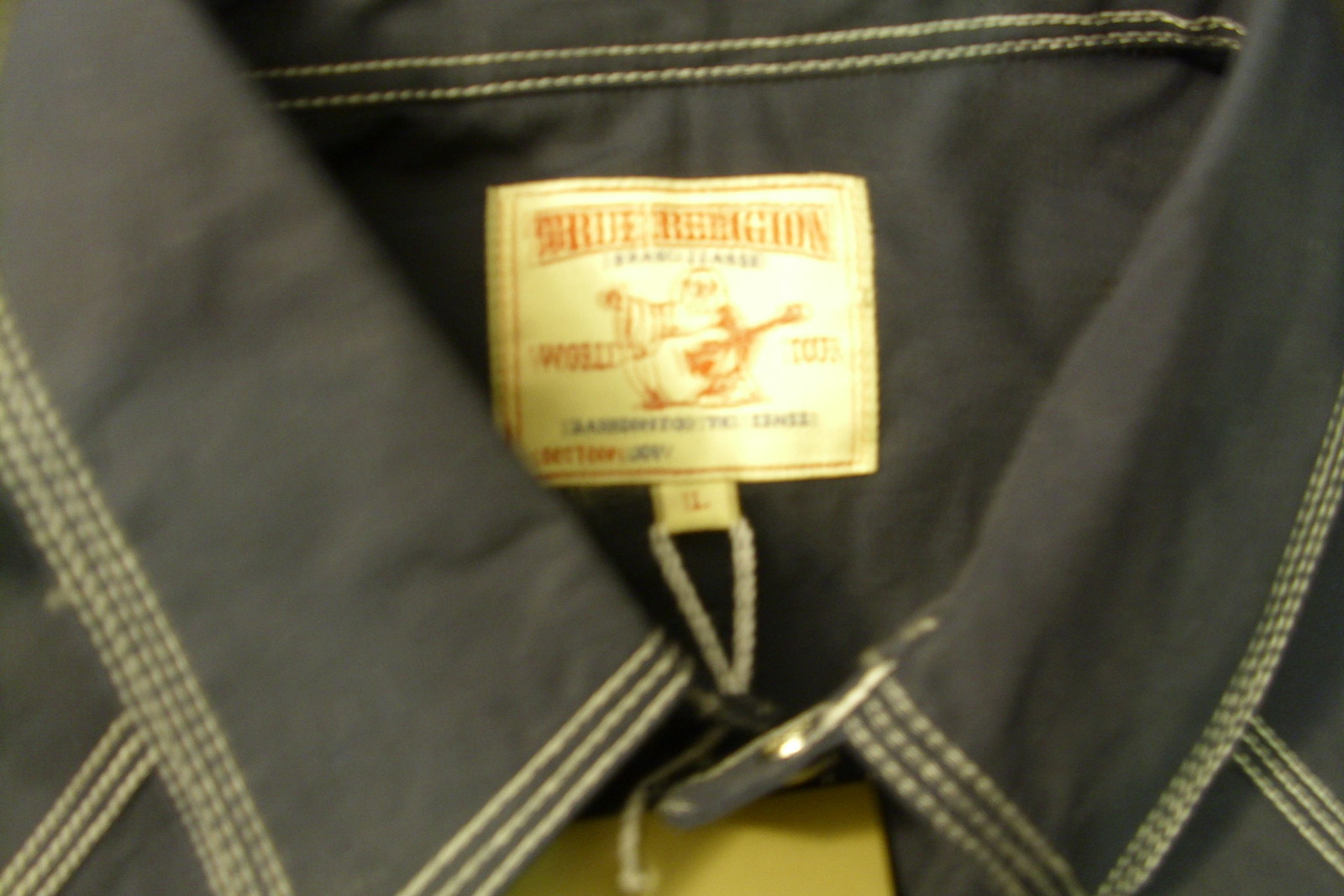A close-up image of a black button-up shirt, focusing specifically on the collar. The fabric of the shirt is black with intricate yellow triple-line stitching that adds a touch of detail to the garment. Inside the collar, a white tag features red lettering, with a prominent red symbol or logo in the center. Beneath this tag, a smaller tag displays more red text. A white string is attached to the collar, tied to which is a small yellow slip of paper, though its inscriptions are not visible. Additionally, there is a metal clip or button on the collar, adding further detail to the accessory's design.